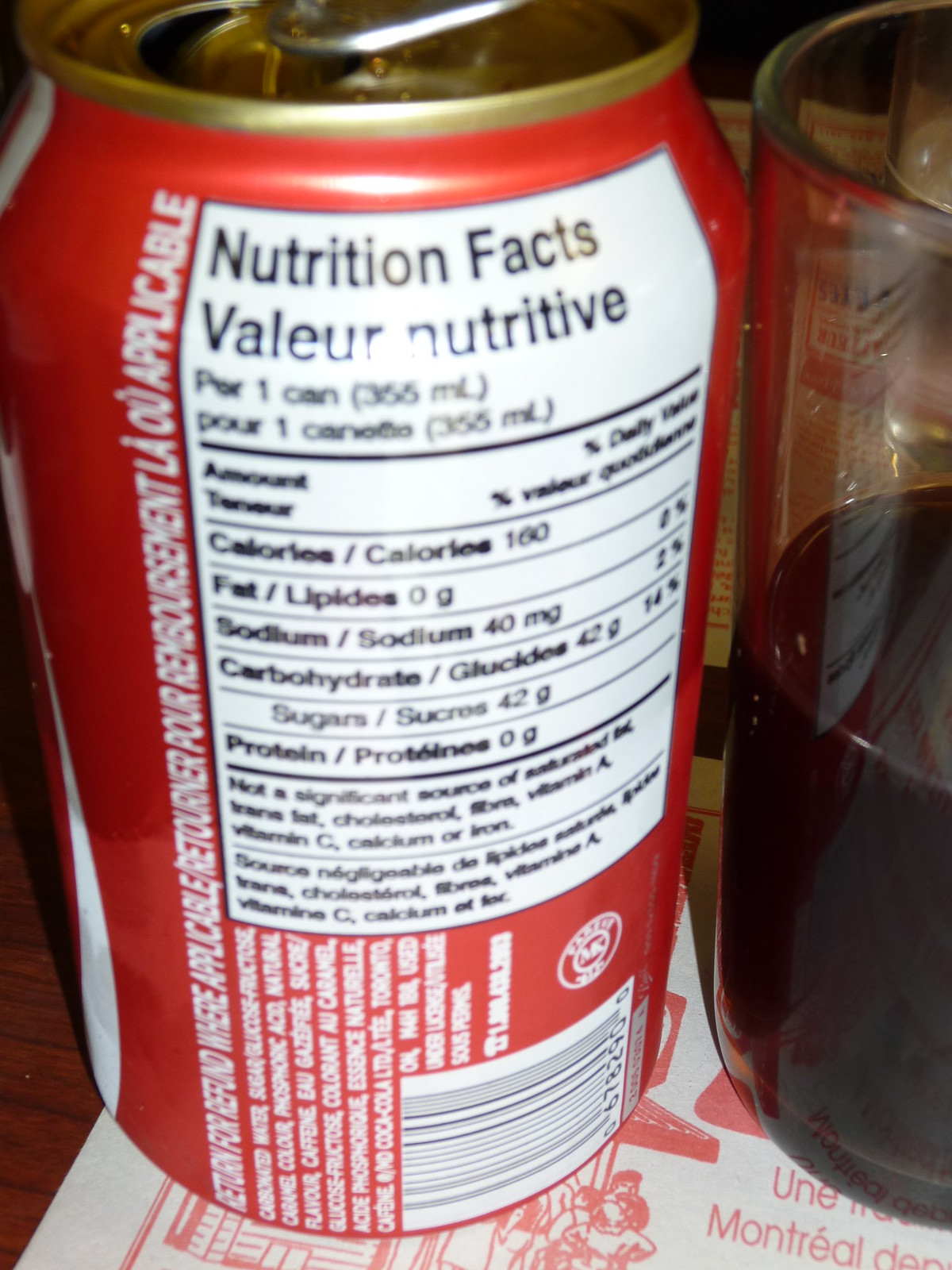This image depicts the detailed nutritional information and labeling for a can of Coca-Cola. Prominently displayed is the standard 'Nutrition Facts' chart, delineating key dietary information in both English and French, indicating its bilingual nature. The label specifies that one can contains 355 milliliters of the beverage. It details the caloric content as 160 calories per serving, and lists essential nutrients such as fat, sodium, carbohydrates, and proteins, alongside their corresponding values. Additionally, it mentions that the product is not a significant source of certain other nutrients, although this part of the text is somewhat unclear. Beneath the nutrition facts, a UPC barcode is visible. Along the side of the label, there is a note regarding can refund policies, though the specifics are difficult to discern. The ingredient list for Coca-Cola is also presented, printed in both languages for wider accessibility.